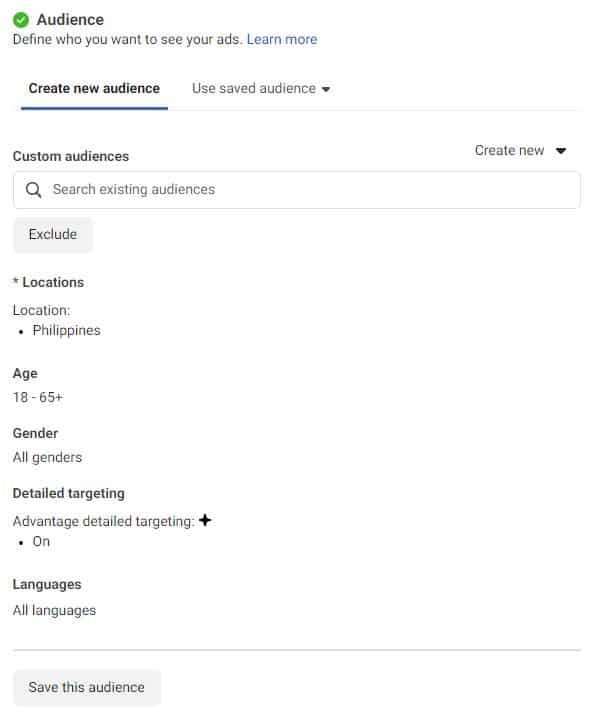This image is a detailed screenshot of an audience targeting form, likely from an advertising platform such as Google Ads, displayed in portrait mode with a predominantly white background. 

In the upper left-hand corner, there's a green checkmark followed by the bold text "Audience." Directly below, the text "Define who you want to see your ads" appears, accompanied by a blue link labeled "Learn More."

The form is divided into two primary tabs, each accessible via dark blue, underlined text. The left tab, which is active, is labeled "Create New Audiences," while the right tab says "Use Saved Audience" with a drop-down arrow for selection. 

The next section begins with the bold label "Custom Audience" followed by the option "Create New" on the right, which also includes a drop-down arrow. Below this, there's a prominent search bar with the placeholder text "Search Existing Audiences." Adjacent to it is a gray button labeled "Exclude."

The form further categorizes the audience parameters as follows:

- **Locations**: The selected location is the Philippines.
- **Age**: The selected age range is from 18 to 65+.
- **Gender**: The setting indicates "All Genders."
- **Detailed Targeting**: Marked by a bold label "Advantage Detailed Targeting," which includes a highlighted plus sign, indicating this option is turned on.

The final section lists "Languages" with the setting "All Languages." 

A thin gray line divides different sections of the form. At the bottom, there's a light gray button that reads "Save This Audience," indicating the action to finalize and save the audience settings.

This form provides a comprehensive set of options for advertisers to refine and define their target audience for campaigns.